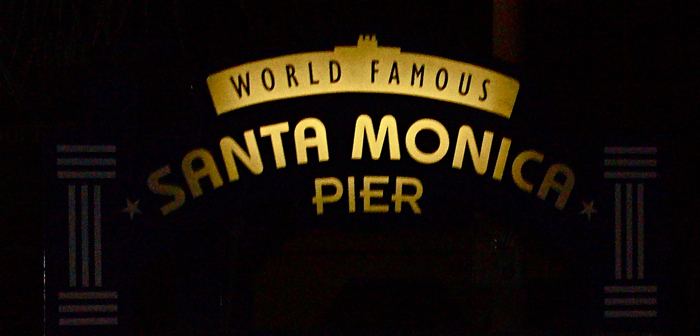The image resembles a cinematic still, featuring a predominantly black background with subtle details emerging upon closer inspection. Dominating the top portion is a gold arched banner with the words "World Famous" inscribed in black, standing out against the gold. Below, in large, bold, gold letters are the words "Santa Monica," flanked by a small star on each side. Beneath this, in gold but less prominent, is the word "Pier." The left and right sides of the image feature vertical symbols that look like columns made up of three horizontal lines at the top, three long vertical lines in the middle, and three horizontal lines at the bottom. These symbols are subtle and blend into the dark background, appearing as a light grayish tone. The entire composition conveys a sense of iconic grandeur, reminiscent of a movie marquee.